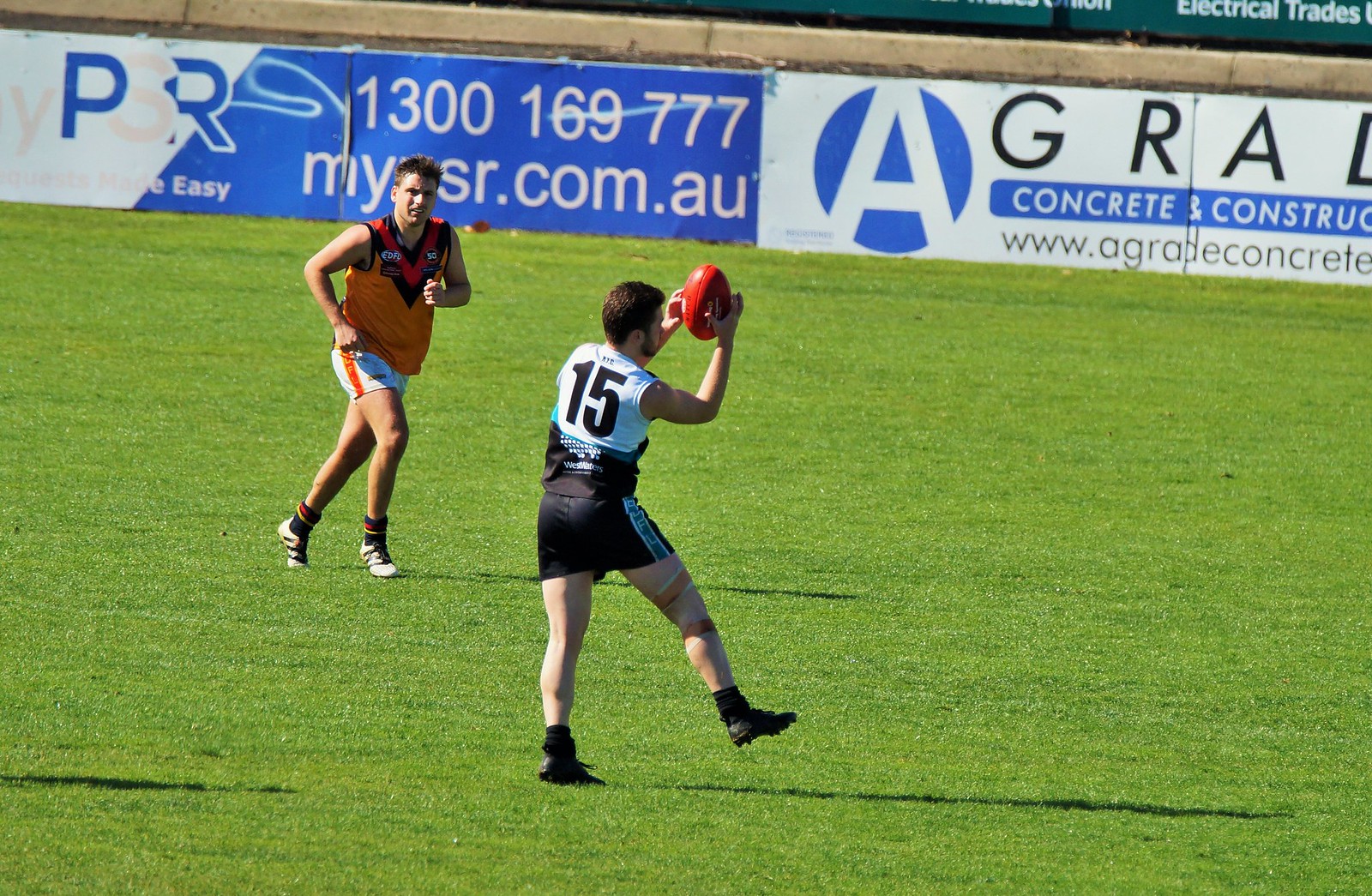The image captures an intense moment on a brightly lit, green rugby pitch where two athletes are the focal point. The main player, wearing a black and white sleeveless jersey numbered 15 and black shorts with a blue stripe on the right side, holds a football as if he has just caught it. He sports black cleats and has a brace on his right knee. Behind him, running in pursuit, is another player dressed in an orange tank top, white shorts, and white cleats. The pitch is meticulously maintained with short-cut grass that radiates a vibrant green hue. In the backdrop, there's a stone fence adorned with advertising banners. One reads "PSR" and "mypsr.com.au," alongside a phone number, "1300-169-777." The adjacent banner, on a white background featuring a blue circle with the letter "A," promotes "A-grade Concrete and Construction" with a partially visible URL, "www.agradeconcrete.com." Shadows cast on the field suggest it's a sunny day, adding to the dynamic energy of the scene.